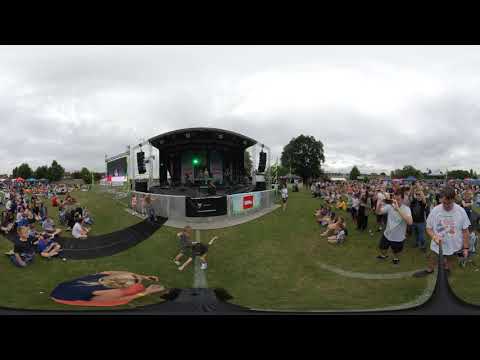This image captures a panoramic, 360-degree view of a bustling outdoor concert festival under an overcast sky. Centrally framed is a stage equipped with various musical gear, flanked by side speakers and a canopy overhead. In front of the stage is a metal barrier. A large crowd, composed of both standing and seated attendees, extends across the scene, with some people seated on grass patches in front of the stage and two young children dancing nearby. Among the crowd, a man in a white t-shirt can be seen on the right side, holding out a selfie stick to capture a wide-angle shot of the event. On the left, there's a significant rectangular screen, mounted on a large metal structure, providing a view of the stage for those further back. Dense, green trees form the background of this lively and varied scene, adding to the vibrancy of the gathering.